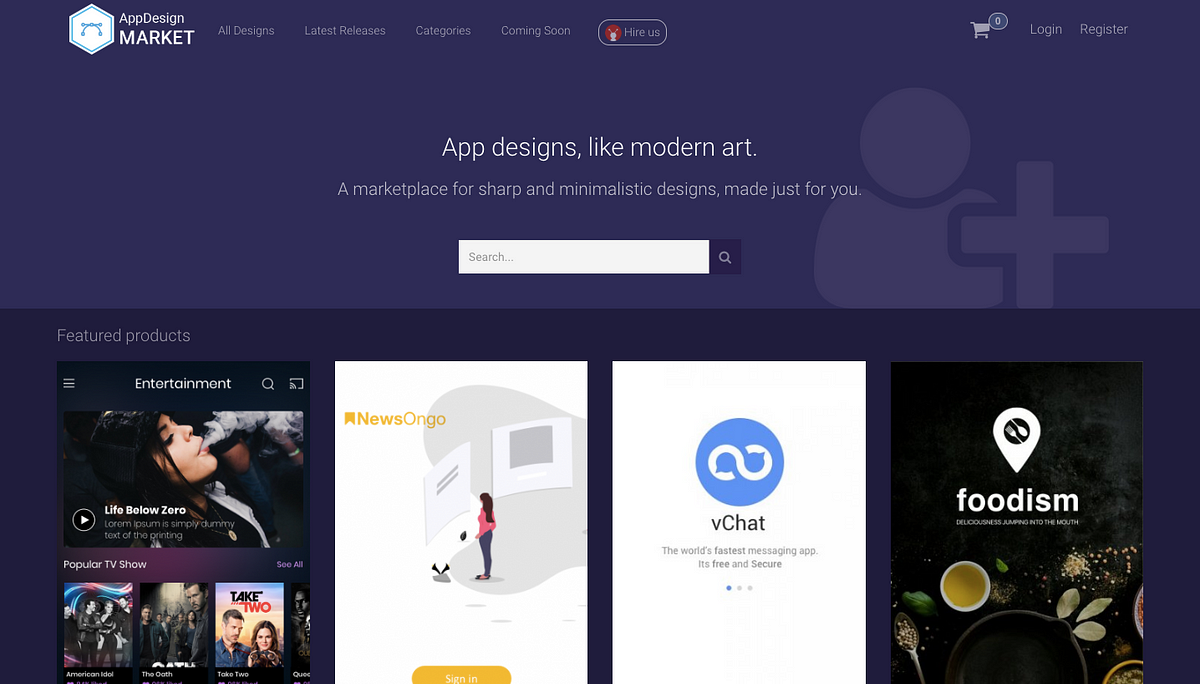The homepage of the website features a dark purple background with a prominent diamond shape positioned in the top left corner. The diamond has a layered appearance with an outer white border, a blue middle border, and a white fill. Inside the diamond, there is an upside-down "U" shape with dots at each end, intersected by a horizontal line with dots at its endpoints. 

To the left of the diamond, in bold, capitalized white text, it reads "APP DESIGN," marked for emphasis. Adjacent to this, in smaller font, the menu options are listed horizontally: "All Designs," "Latest Releases," "Categories," "Coming Soon," and "Hire Us." The "Hire Us" option is enclosed in a white border and is accompanied by a small, gray robot icon and a red circle to its left. 

On the right side of the top menu, you find small text for "Register" and "Log In," followed by a shopping cart icon with a circle displaying a "0" inside it.

Centrally positioned beneath "Hire Us," about two inches down, the text "APP DESIGNS" is followed by a comma, then "LIKE MOD OR NOT." Underneath this header, a tagline reads "A marketplace for sharp and minimalistic designs, made just for you," in smaller white lettering.

A white search bar is positioned underneath the tagline, with placeholder text "Search" inside it. On the right of the search bar, there is a darker purple square containing a white search icon.

Below the search bar, on the left side, the heading "FEATURED PRODUCTS" appears in white text. Underneath this heading, four rectangular sections are aligned horizontally. The first rectangle, labeled "ENTERTAINMENT," features an image of a woman blowing out smoke and is a preview for a video titled "Popular TV Show." 

The second rectangle showcases an image of three TV shows with a white square labeled "NEWS ON GO" in the top left corner, depicting a drawing of a woman in the center and a yellow tab labeled "SIGN IN" at the bottom. The third rectangle, set against a white background, includes a blue circle with a sideways "S" and is labeled "VChat" with two lines underneath it. The fourth rectangle features a black background with a location-like icon encasing a white spoon and fork, labeled "FOODISM." Sprinkles, bowls, and plates are scattered at the bottom.